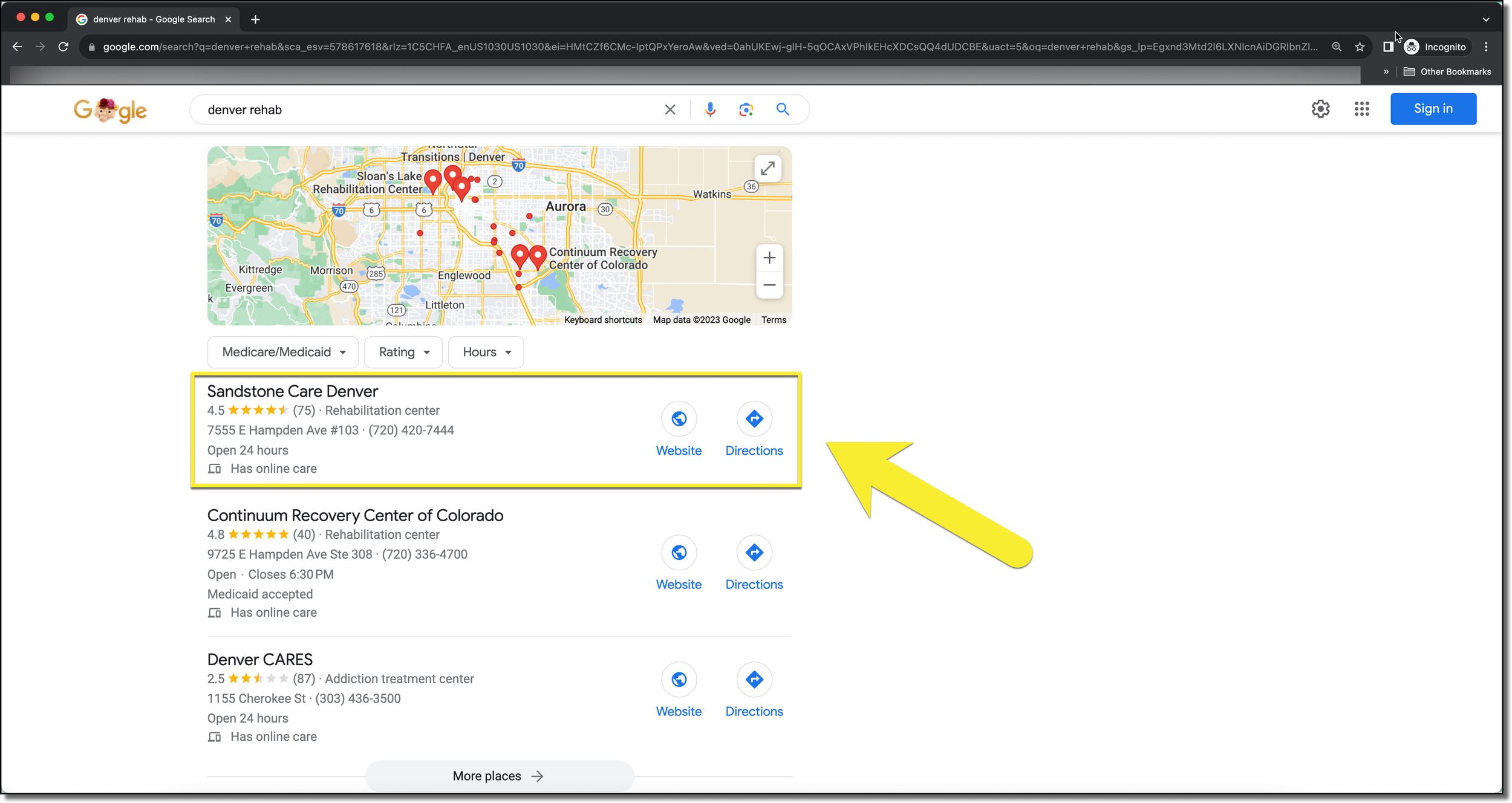The image reveals a Google search query for 'Denver Rehab' on a macOS device. The screen displays the Google search results page scrolled down to showcase a map and list of rehabilitation centers in Denver. The first result, 'Sandstone Care, Denver', is conspicuously annotated with a yellow rectangular highlight and an arrow pointing towards it. The second search result is 'Continuum Recovery Center of Colorado', and the third one is 'Denver Cares'. At the top of the list, a map illustrates multiple rehabilitation locations, while a 'More places' icon is visible at the bottom of the map. The user performing the search hasn't signed into their Google account; consequently, a generic interface is displayed. Each listed location on the map includes options for visiting the respective website or obtaining directions.